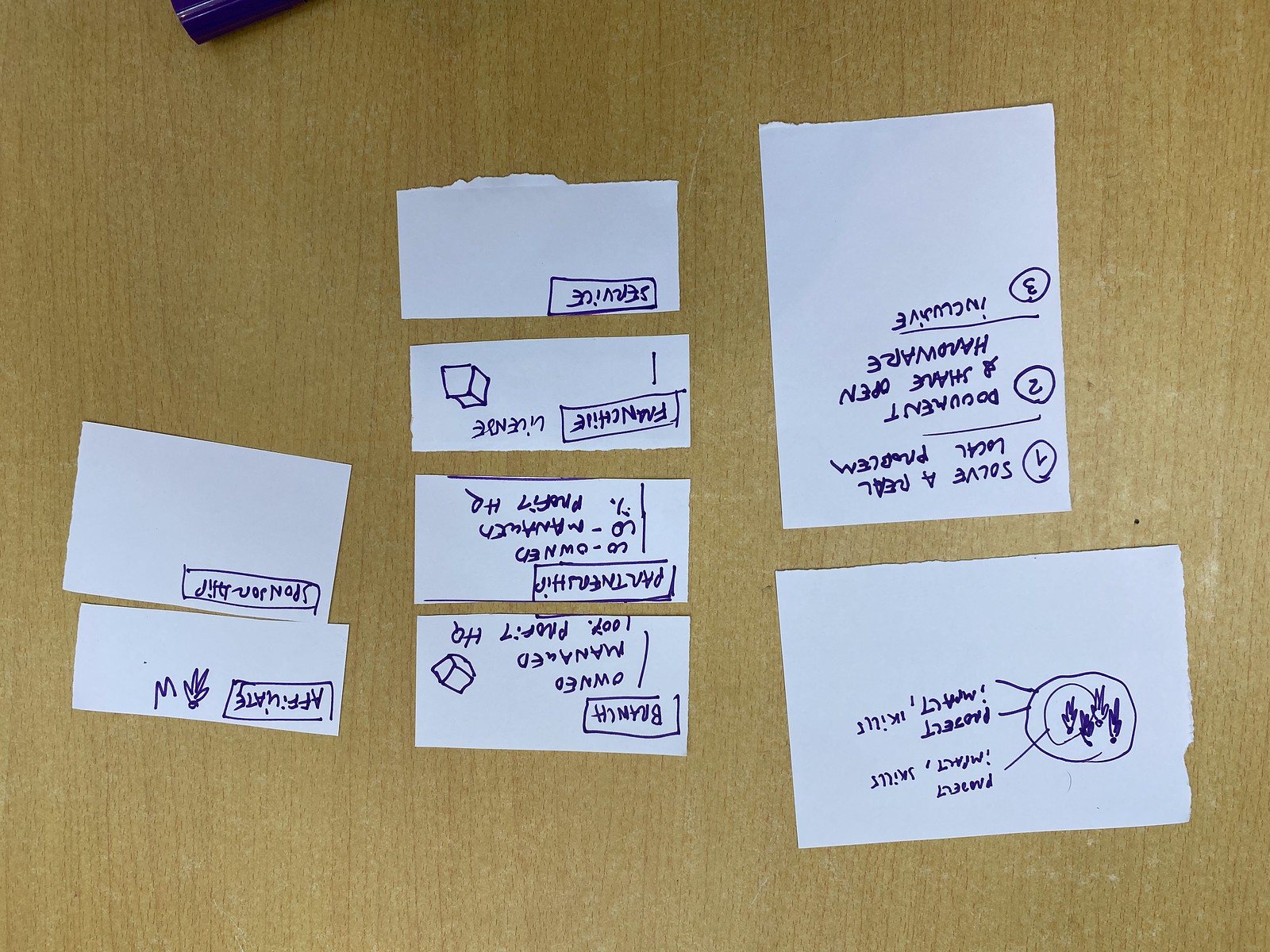The photograph captures a scene of a light oak wood table scattered with various pieces of paper, each marked with detailed, handwritten notes in purple marker. On the left side of the table, two small, cut pieces of paper can be seen. The first one bears the word "affiliate," while the second reads "sponsorship."

In the center of the table, four small rectangular pieces of white paper are arranged in a vertical column:
- The lowest rectangle has the words "branch," "owner," "manager," and a partially obscured phrase ending in "headquarters."
- The next rectangle up contains the word "partnership" and some illegible text.
- The third rectangle displays the word "franchise" and features a small, 3D box drawing.
- The topmost rectangle simply says "service."

All the words on these papers are framed within neatly drawn squares.

On the right side of the table are two larger rectangular pieces of paper, one oriented horizontally and the other vertically. 
- The lower rectangle features a crude drawing of several people in a circle, surrounded by additional words related to "skills" and "IT protection," though these texts are upside down.
- The upper rectangle contains a numbered list:
  1. "Solve a real local problem"
  2. Includes partially legible phrases such as "document and share open hardware."
  3. Conveys ideas related to "income" or "inclusive."

This detailed arrangement suggests a brainstorming session or organizational planning process, with each piece of paper representing key concepts or elements within a larger strategy.